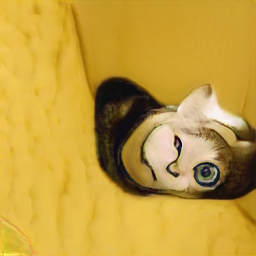This square, photographic image possesses a surreal, almost abstract quality, depicting a cat indoors with striking, unusual features. Set against the majority of a mustard yellow background, with varying shades and textures, the cat sits in the corner of a yellow sofa. The feline’s right eye is large, green, and surrounded by a stark black outline, while its left eye appears squinted and obscured by its cheek, giving the face a distorted appearance reminiscent of Picasso-esque art. The cat’s black fur is intermixed with patches of grey, brown, and white, and it has two visible ears, the top left ear appearing disproportionately larger due to the angle. A black line is present beneath the cheek, enhancing the surrealism. Though its body lacks discernible features such as legs or a tail, the unusual composition unmistakably forms a cat's face.